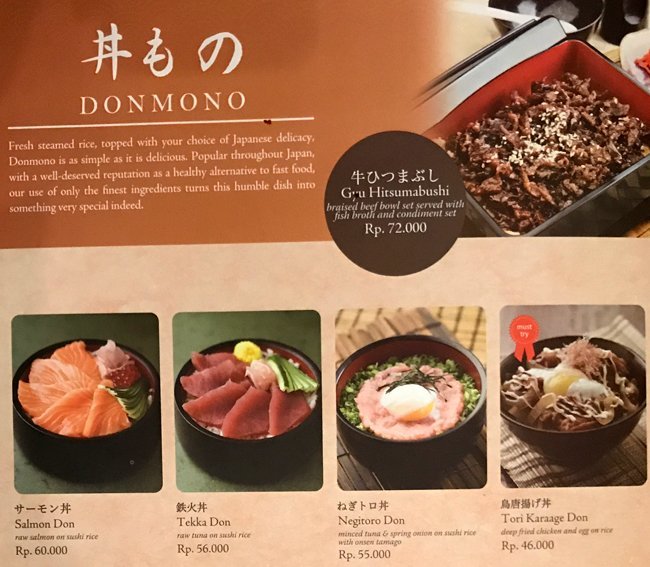The image features a wide rectangular section of a menu, primarily beige and light caramel brown in color. Dominating the upper left corner, white text on the caramel background reads "Don Mono" in all capital letters, accompanied by three Japanese characters. Below this, a white line separates the title from a descriptive paragraph in white text that emphasizes the simplicity and deliciousness of Don Mono, highlighting it as a popular and healthy Japanese dish made with the finest ingredients. 

On the upper right side, the caramel hue fades into an enticing image of a beef Asian dish served in a distinctive red and black square-shaped bowl. The menu also showcases four square-shaped images of different Japanese dishes against a beige background, each with a title: Salmon Don, Tekka Don, Negitoro Don, and Torikurage Don. The prices for the dishes are indicated in a currency that appears to be rupees, denoted by "RP" followed by the respective amounts. The menu leans heavily on the theme of authenticity and quality, positioning Don Mono as a healthier alternative to fast food, celebrated across Japan.